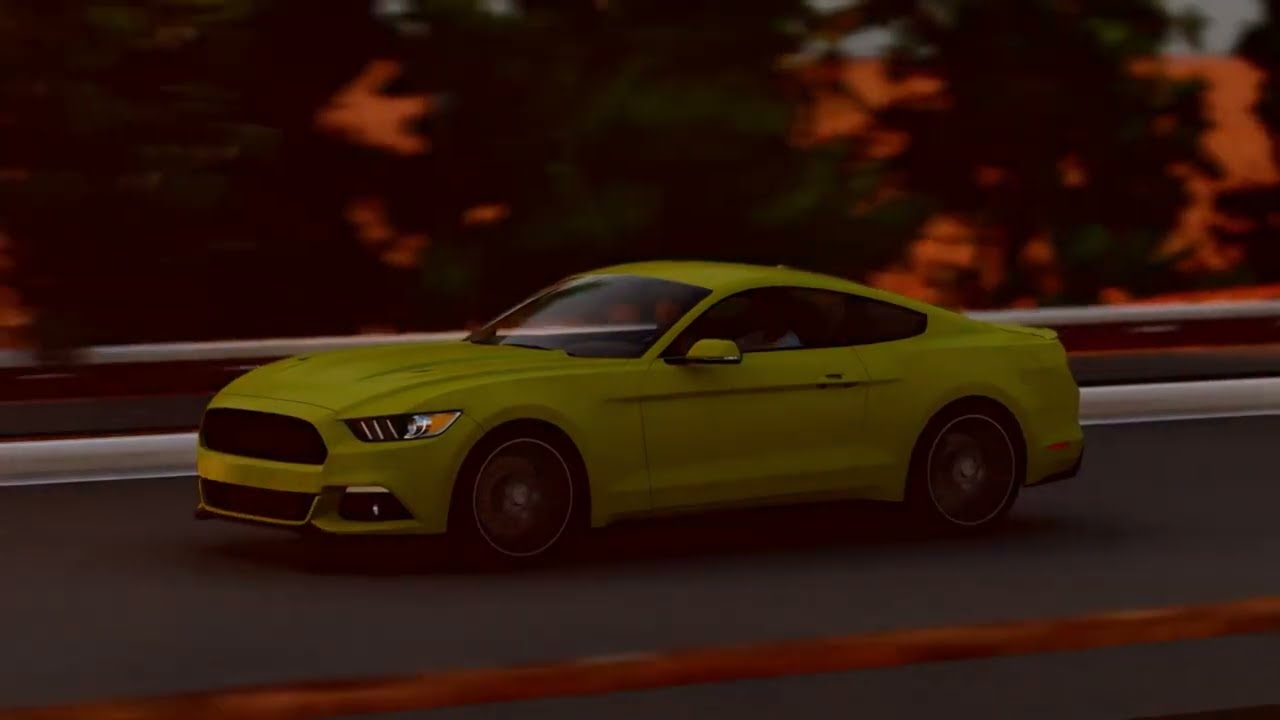This image features a neon lime green or dark yellow Mustang two-door sports car driving on a freshly paved, dark asphalt road, likely a freeway. The car is positioned with its back part to the right and the front to the left, giving the impression of motion. Its sleek, sporty design is accentuated by the noticeable absence of a front license plate and the bright headlights shining from the front bumper. In the distance, there's a white and brown guardrail running parallel to the vehicle. The blurred background hints at orange-hued trees and possibly residential buildings with peeking rooftops, suggesting the road might be elevated. The setting is quite dark, enhancing the car's vibrant color under minimal lighting, and a faint line of orange or red at the bottom of the concrete road adds a subtle contrast. This detailed scene could serve as an advertisement for a new Mustang model due to its striking appearance and realistic, albeit slightly artificial, look.